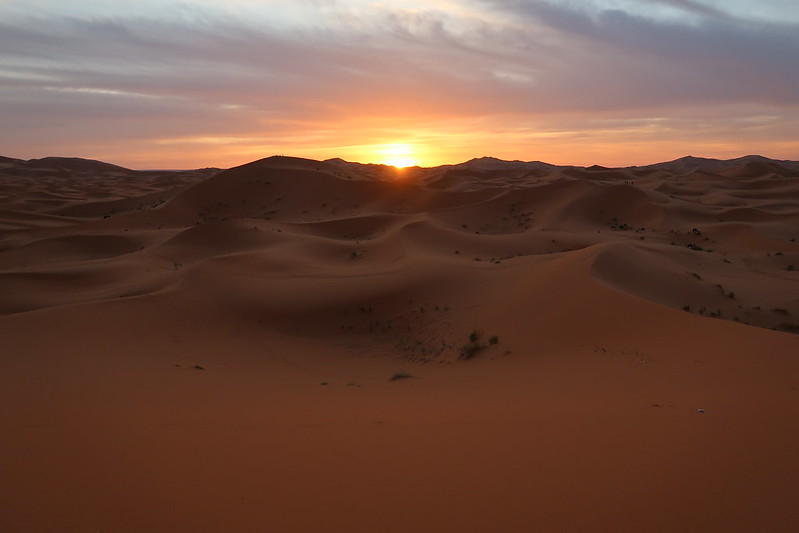A mesmerizing photograph captures the peaceful beauty of a desert landscape at sunset. The scene features flowing sand dunes extending out to a hilly horizon, bathed in a brownish-orange hue from the setting sun. The intricate ripples on the sand add texture and depth to the dunes, interlocking gracefully across the landscape. Sparse desert plants dot the dunes, adding touches of life to the otherwise barren vista. The sun, a glowing orb of white tinged with hints of orange and red, sits directly on the horizon at the center of the photo. Above, a sky painted in shades of gray, dull lilac, gold, and orange creates a magical canopy. The ethereal, cloudy sky enhances the tranquil and natural beauty of the scene, making it a serene and captivating moment frozen in time. No animals or humans are present, leaving the viewer to fully appreciate the undisturbed splendor of the desert sunset.